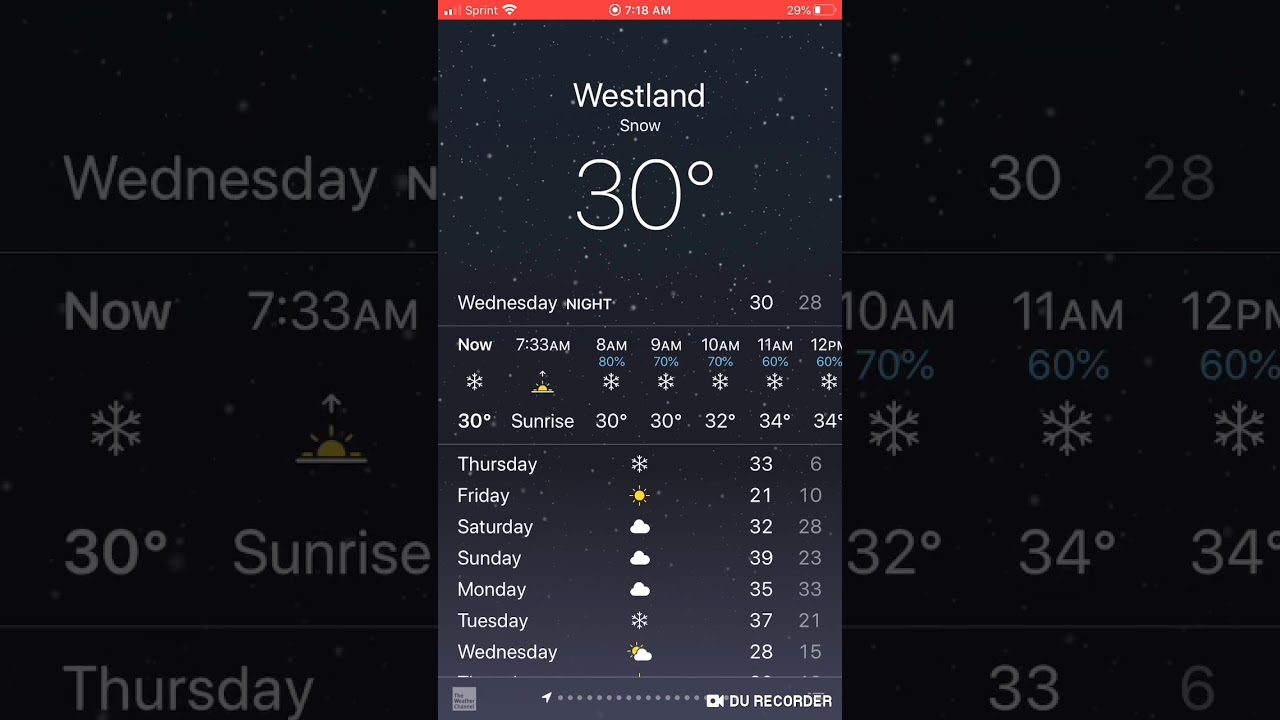This image is a screenshot from a smartphone displaying a detailed weather report for Wednesday in Westland. The timestamp at the top reads 7:18 AM, showing the current snowy conditions with a temperature of 30 degrees Fahrenheit. Below is the forecast for the day and the upcoming week:

- **Wednesday Morning:** 
  - 7:33 AM: Snowing, 30°F
  - 8:00 AM: Sunrise
  - 9:00 AM: 80% chance of snow, 30°F
  - 10:00 AM: 70% chance of snow, 32°F
  - 11:00 AM: 60% chance of precipitation, 34°F
  - 12:00 PM: 60% chance of precipitation, 34°F

- **Wednesday Night:** 
  - High of 33°F, low of 6°F
  
- **Upcoming Days:**
  - **Friday:** Sunny, high of 21°F, low of 10°F
  - **Saturday:** Cloudy, high of 32°F, low of 28°F
  - **Sunday:** Cloudy, high of 39°F, low of 23°F
  - **Monday:** Cloudy, high of 35°F, low of 33°F